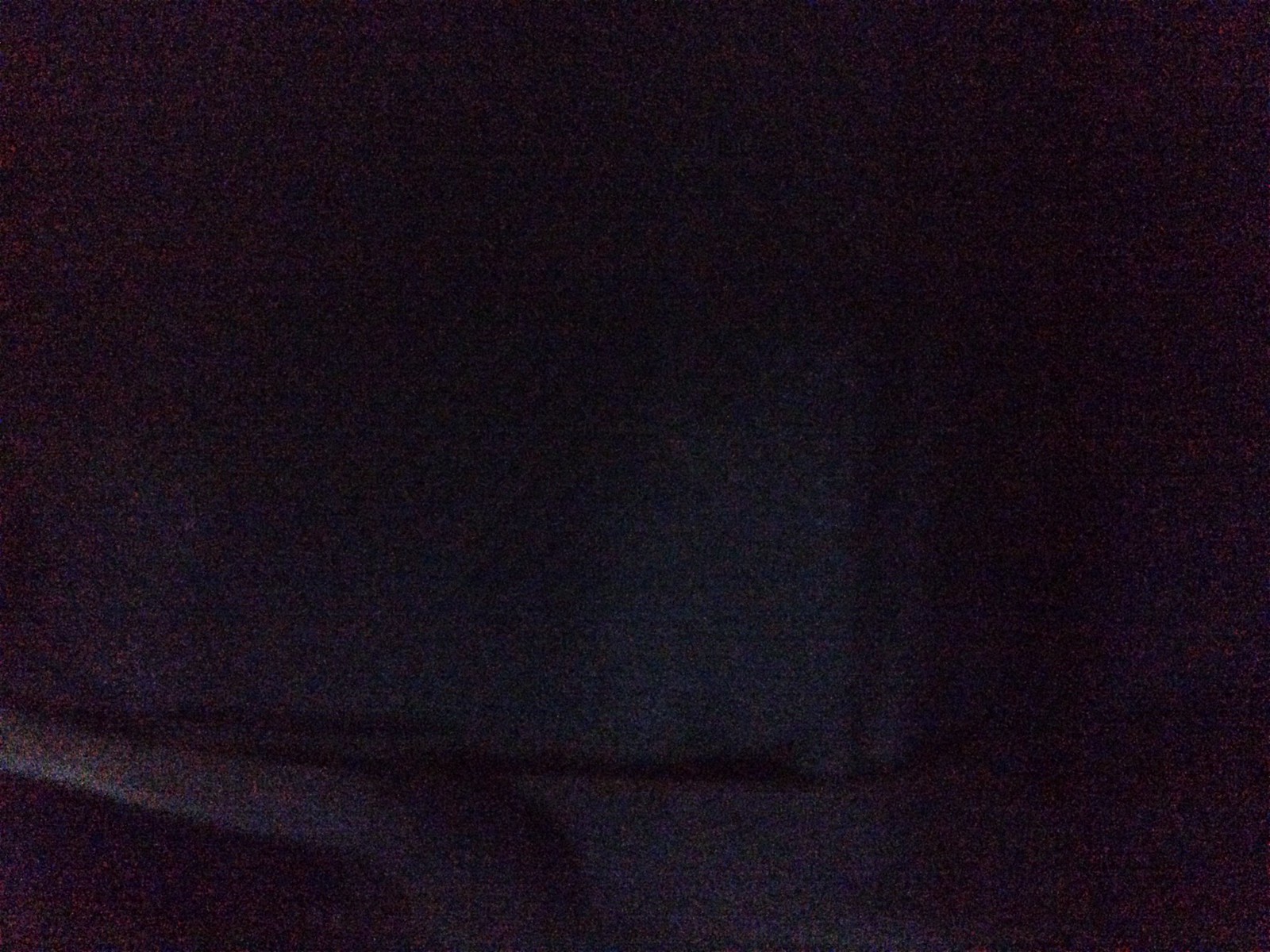This is a photograph taken in an extremely dark and poorly lit room, leading to a very grainy and pixelated appearance. The image is predominantly black, making it almost impossible to discern specific details. Toward the center, there is a faintly visible rectangular or square area that appears slightly lighter in shade, with hints of gray and possibly blue hues. This central object could resemble a window or a poorly outlined structure due to its shape. The top left and right portions of the image remain entirely black, with no discernible features. In the bottom left, there appears to be a rounded shape that might be the back of a piece of furniture, but its exact nature is unclear due to the darkness. Overall, the photograph captures a vague and indistinct scene dominated by darkness and shadow.